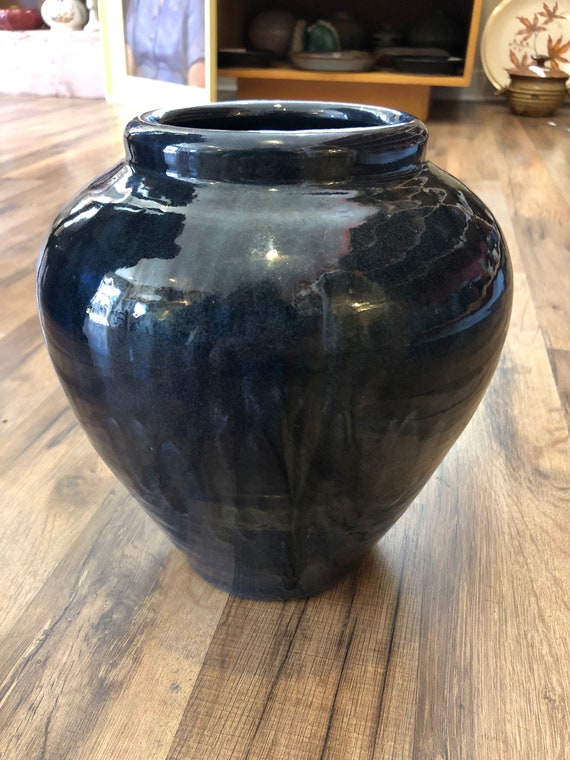The photograph captures a detailed view of a glossy black and gray ceramic vase, prominently positioned in the center of a wood-floored room with a barn-style aesthetic. The vase, which could serve as a jug for holding water or as a decorative piece for dry plants, features a smooth, clear coating enhancing its shiny surface. The robust and sturdy vase is roundish with a smaller point at the bottom, measuring approximately 10 inches high and 8 inches wide. Behind the vase, an open cabinet reveals other ceramic pottery, including a plate with brownish leaf designs and possibly a framed photograph leaning against the wall. The setting further includes an entertainment center adorned with various items such as a round glass object with a plant, contributing to the warm, rustic interior ambiance. There is no text in the image, ensuring the focus remains on the vivid details and composition of the scene.